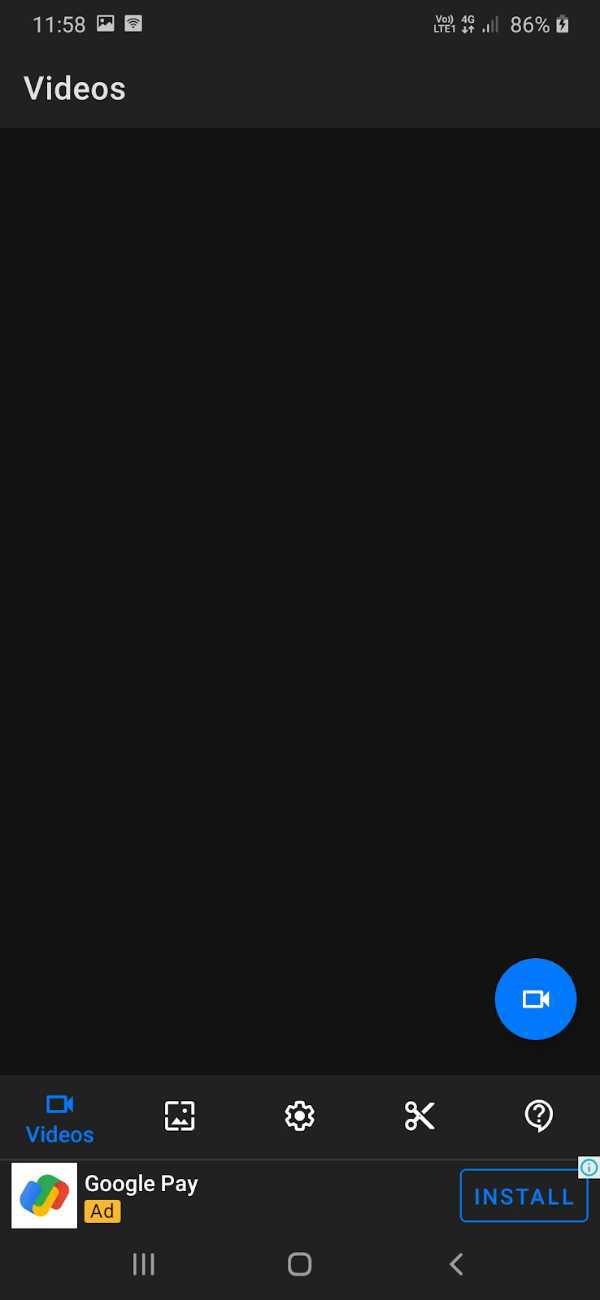This image depicts a mobile application interface primarily dedicated to video management. At the top edge of the screen, the status bar displays essential information including the time (11:58), a Wi-Fi signal icon, a cellular signal bar indicator, and the current battery level at 86%. Below the status bar, the majority of the screen is dark, suggesting either a lack of access to videos or an initial setup phase.

In the middle of the screen, there is a prominent blue button featuring a video camera icon, likely for recording or uploading videos. At the bottom of the main area, a navigation bar highlights the "Videos" tab in blue, emphasizing that this section is currently active. Accompanying this tab are several icons: a picture icon, a settings gear wheel, a pair of scissors with an open handle, and a question mark encircled.

Above the navigation bar, an advertisement for Google Pay is present, marked as an "ad" in yellow with an "Install" button.

Further details are found at the bottom edge of the screen, where there are three additional buttons: a three-line menu icon, a central circular button, and a right-pointing arrow, presumably for navigating or performing additional actions.

The image combines dark and light elements, with most of the screen being black contrasted by white text and vibrant icons, suggesting either restricted access to content or an uninitialized app screen on a new device.